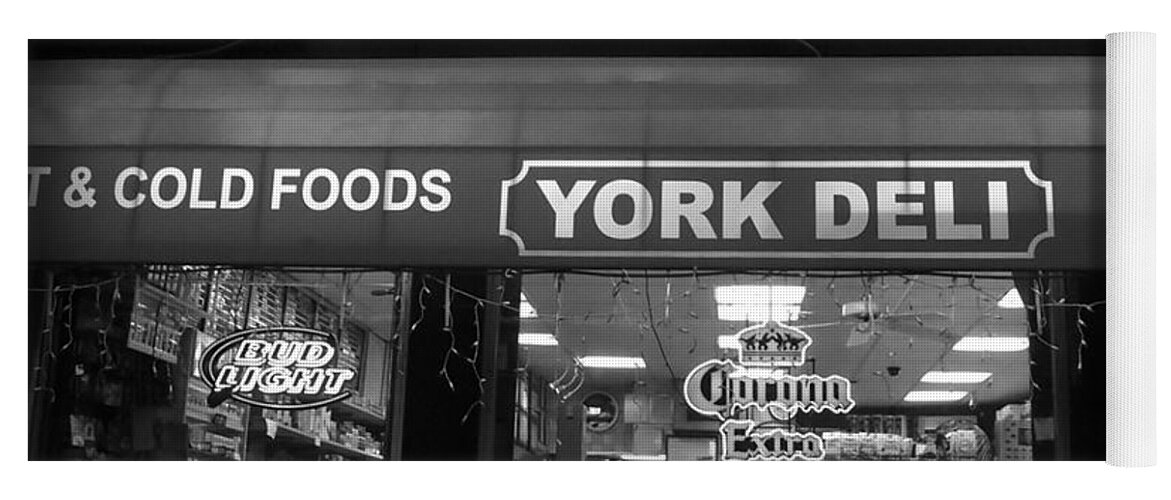This detailed black and white photo captures the exterior and partial interior of a New York deli at night. Dominating the scene is the storefront, featuring a large sign reading "York Deli" in bold white text on a bordered banner prominently displayed above the right-hand window. Adjacent to this sign, the words "Hot and Cold Foods" are partially visible, showing only "Cold Foods" clearly. Below these signs, the left window displays a bright Bud Light neon sign, while the right window features a Corona Extra neon sign. Through the glass, the interior ceiling is visible, adorned with old-fashioned tiles, panel fluorescent lights, and at least two surveillance cameras. Exterior Christmas lights hang from the ceiling outside, adding festive decor to the scene. On the far left, a glimpse of the interior wall reveals a display of various foods and snacks, under the glow of the deli's interior lighting.